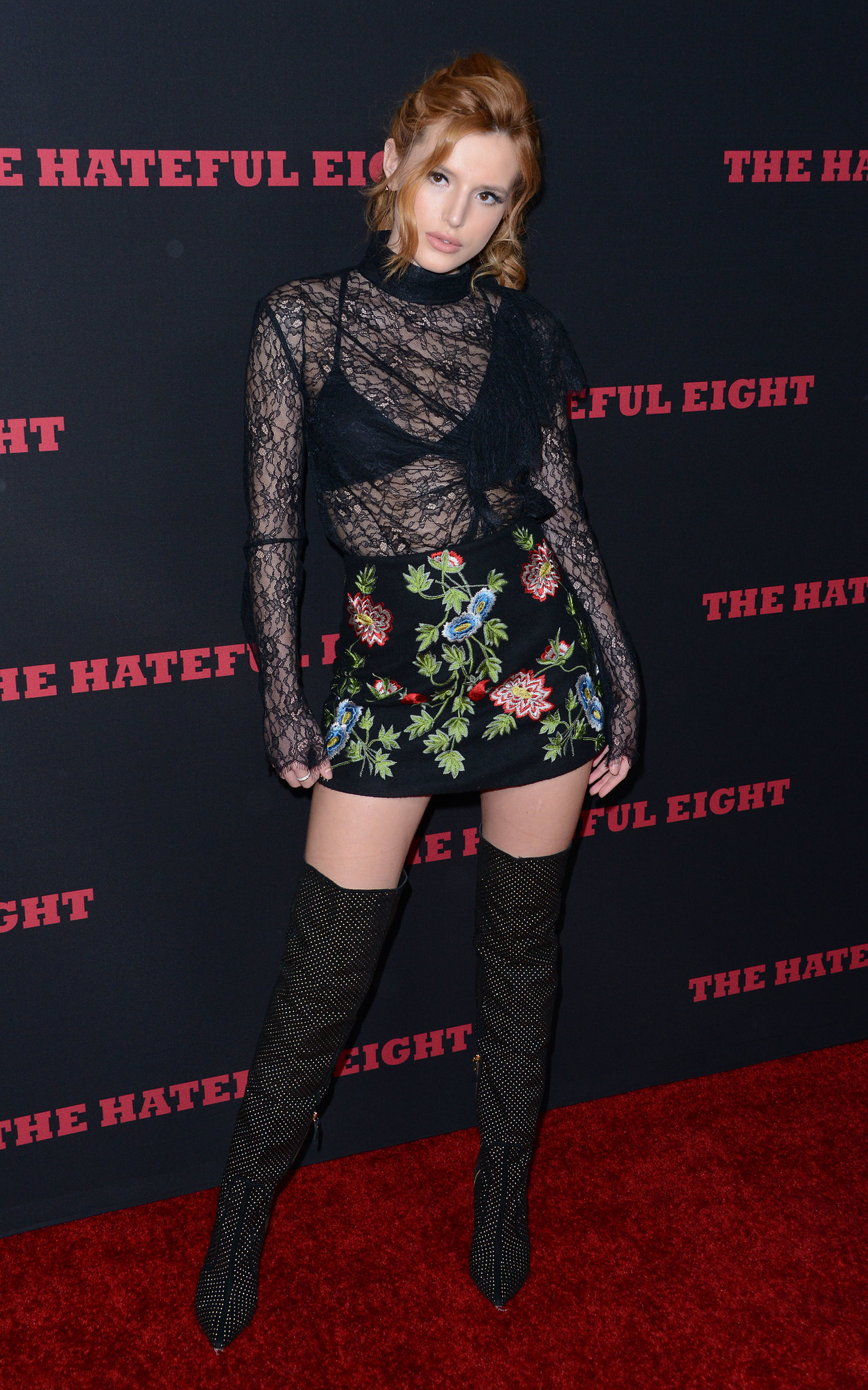A young, attractive actress is posing on a blood-red carpet at the presentation of the movie "The Hateful Eight." The photo captures her standing indoors in front of a black wall covered in red lettering that repeatedly spells out "The Hateful Eight." She is of Caucasian descent and has reddish hair pulled back, with long tendrils framing her face, which notably features pink lipstick and a straight nose. Her head is tilted to one side, and her hips follow the same tilt, creating a striking pose. She is dressed in a black lace long-sleeve top that is see-through and extends to her fingertips, revealing a black bra with fringe on one side underneath. She pairs this with a short black mini skirt adorned with bright floral patterns—green leaves and pink and blue flowers. Completing her outfit are tall, thigh-high black boots embellished with white dots. Her overall ensemble highlights her trim figure and exudes a chic, fashionable vibe suitable for the event.